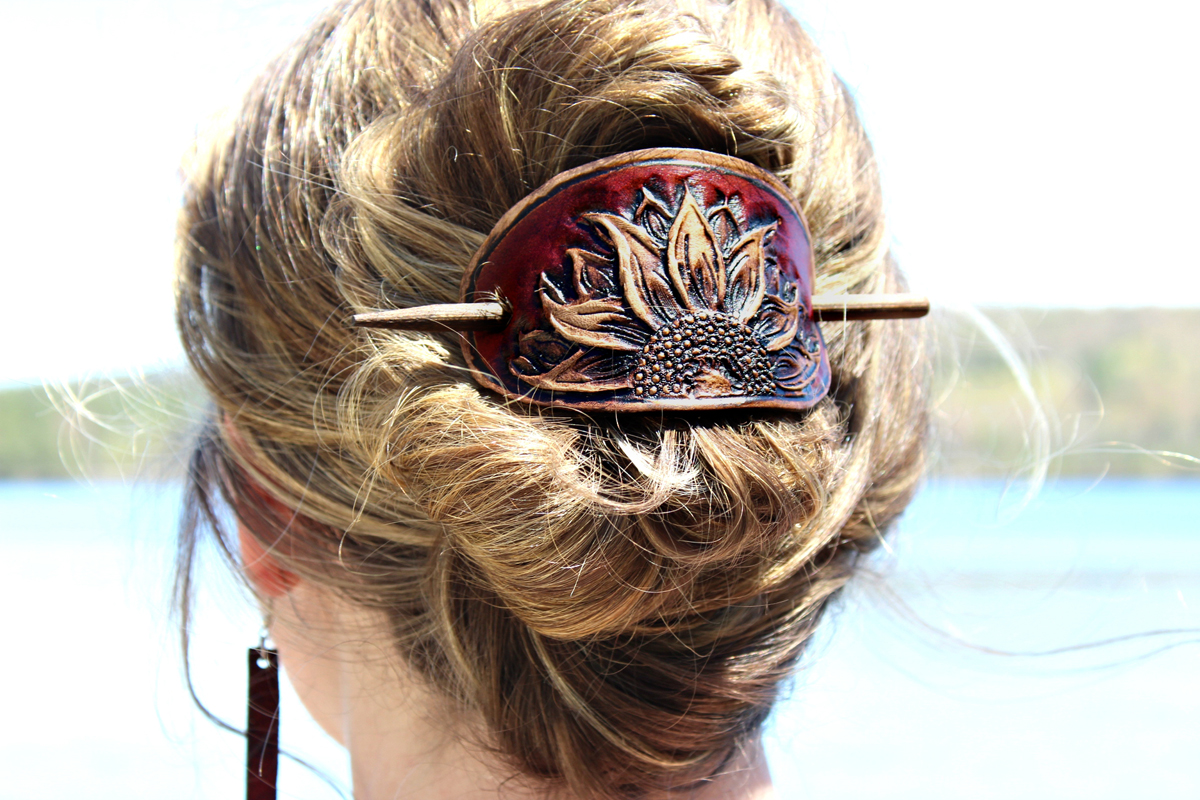The photograph captures the back of a woman's head, showcasing her dirty blonde hair with subtle blonde highlights, styled in a messy bun. Her hair is secured with an elegantly ornamental leather barrette, which features an embossed design of half a sunflower, with lighter-colored petals contrasting against a darker brown background. A tan-colored stick, resembling a pencil, holds the barrette in place. Visible on her left ear is a long, rectangular dangling earring. The background of the photo is softly blurred, revealing hints of blue water, greenery, and a bright, white sky, suggesting an outdoor setting on a sunny day. The woman’s light complexion hints at a possible North European heritage.